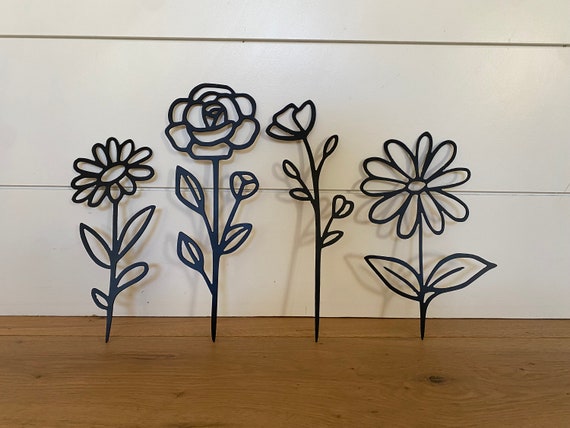The image captures an indoor art installation featuring an arrangement of metallic flower sculptures, crafted from a hard, dark metal, possibly wrought iron. These sculptures are propped against a pristine white wall, set atop a well-polished, laminated wooden floor. The collection includes realistic representations of various flowers such as a rose, a tulip, and two daisies, characterized by their distinctive petal formations and stems of varying lengths. Each flower has two to four leaves extending from its sides, and they collectively cast elegant shadows on the white wall behind them, adding depth to the scene. The tallest sculpture is the rose, followed by the tulip, with the two daisies being approximately the same height but differing in petal and center size. The overall setting presents a harmonious blend of art and nature, combining intricate metalwork with the serenity of floral imagery.